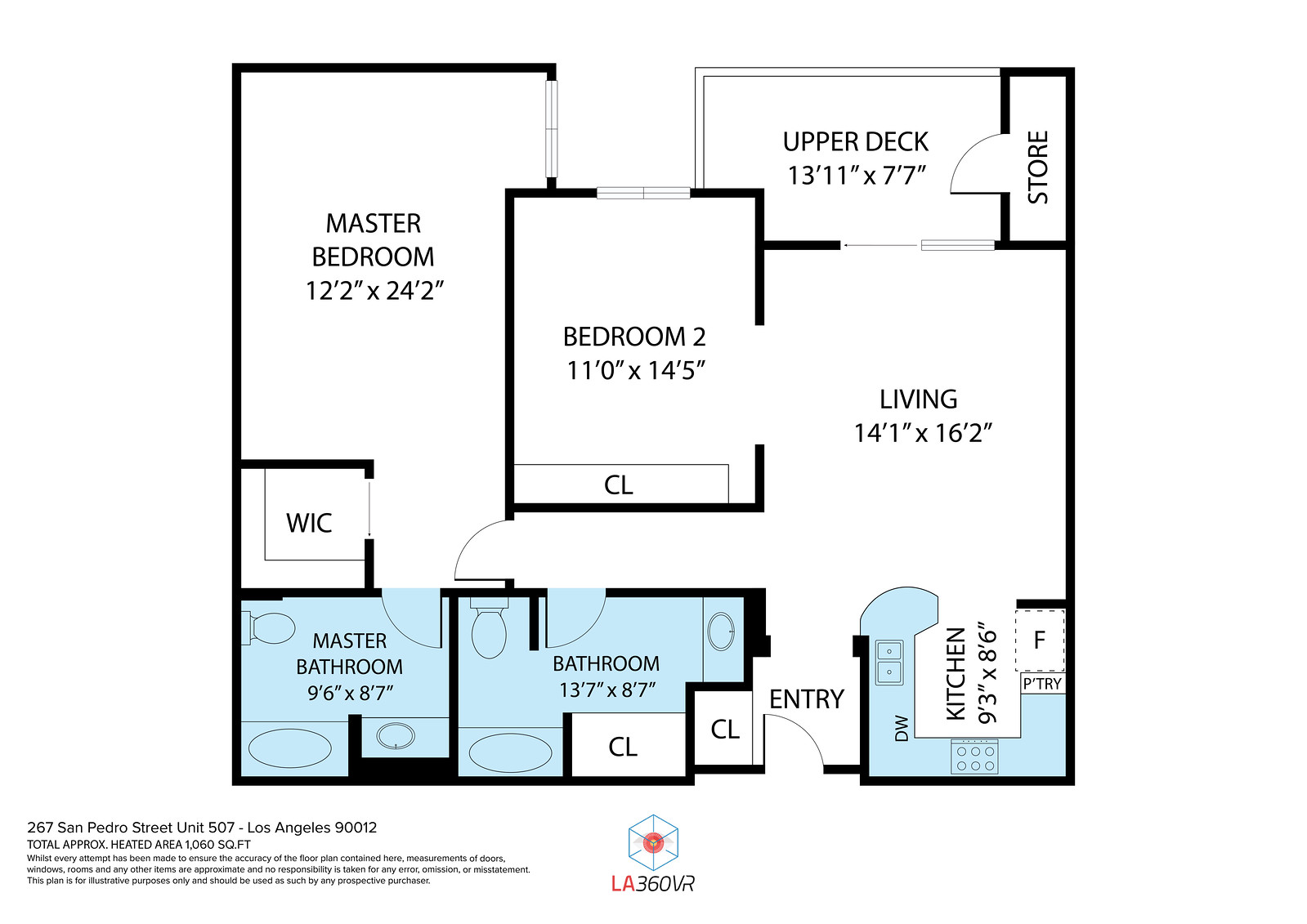This is a color digital floor plan with a roughly square shape, meticulously divided into various rooms. 

- **Upper Left Corner**: The master bedroom, labeled in uppercase black letters, measures 12 feet 2 inches by 24 feet 2 inches.
  
- **Center**: Bedroom 2 is centrally located, enclosed by black borders, measuring 11 feet 0 inches by 14 feet 5 inches. A small rectangular space at the bottom of the room delineates a closet.

- **Upper Right Corner**: Here lies the upper deck, which includes a labeled storage area ("Store").

- **Middle Right**: The living area, labeled "Living," measures 14 feet 1 inch by 16 feet 2 inches.

- **Lower Right Corner**: The kitchen area, highlighted in light blue, is situated here. Immediately to the left of the kitchen is the entry area.

- **Left of Entry**: Adjacent to the entry area is a bathroom, also filled with light blue color.

- **Bottom Left Corner**: The master bathroom is positioned here.

Additionally, in the bottom-left corner of the floor plan, two pieces of information are provided in black letters:
- The address: 267 San Pedro Street, Unit 507, Los Angeles, CA 90012.
- Total approximate heated area: 1,060 square feet.

This descriptive arrangement ensures clarity and detail for each part of the floor plan.